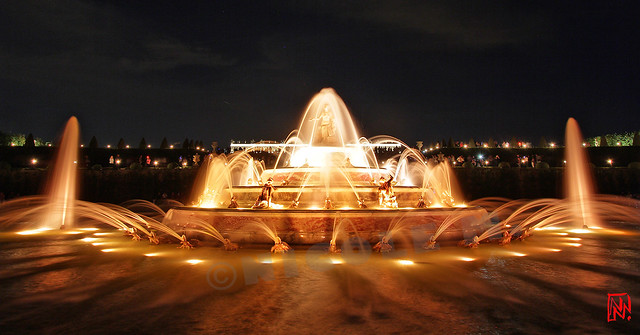The photograph captures a grand, ornate fountain illuminated against a pitch-black night sky, creating a mesmerizing golden glow. At the center of the fountain stands a prominent statue of a man, surrounded by various other statues, including two men reaching toward the sky near the bottom level. Multiple tiers of the fountain ascend like a multi-layered cake, each adorned with intricate sculptures, including fish with their mouths open, spraying water. The outermost ring features fish sculptures facing outward, shooting streams of illuminated water into a large surrounding pool or moat. Vertically upward streams of water on either side add to the dynamic display. The water appears misty and slightly out of focus due to a time-lapse effect, enhancing the ethereal quality of the scene. In the bottom right corner, a black and red watermark with an upside-down "W" or "M" is visible. The night sky is deep and dark, with silhouetted trees lining a wall in the background, complemented by distant lights that hint at a cityscape beyond.